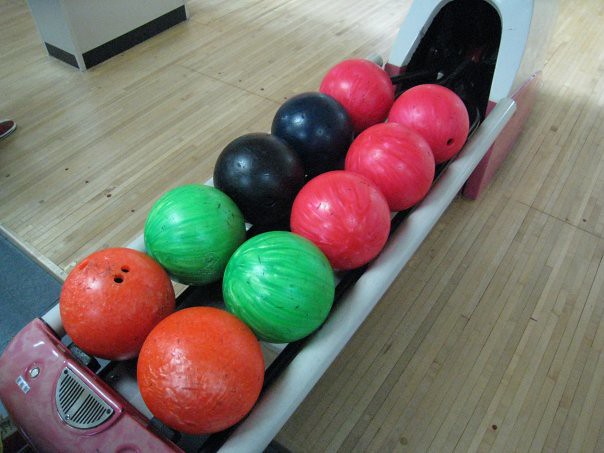This image captures a detailed scene at a bowling alley. The floor is composed of long, thin strips of light brown wood, characteristic of a typical bowling alley. Diagonally across the image, from the bottom left to the top right, runs a white and dusty red ball return dispenser. It features white rails and holds ten bowling balls. The bowling balls are meticulously lined up with two orange balls at the closest point to the camera, followed by two green ones, two black and pink ones, and four pink ones positioned furthest away. To the left edge of the image, the wooden floor transitions to a dark grayish-blue carpet, which marks the seating area for players. Additionally, the upper left corner reveals part of a support pillar and a glimpse of someone’s shoe.